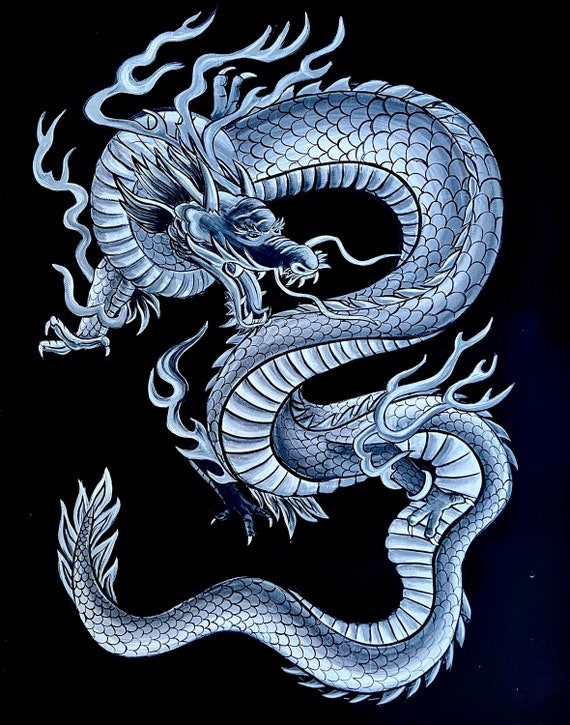The image depicts a detailed illustration of a Japanese-style dragon set against a pitch-black background. The dragon is long and slender, its sinuous body coiling across the entire image, giving it a dynamic, almost floating appearance reminiscent of traditional Chinese dragon depictions. The dragon's design exudes an ancient yet modern tattoo aesthetic, entirely rendered in varying shades of blue. It features sharp, open teeth and blazing eyes, exuding an angry expression. Horns extend from its head, accompanied by mustache-like antennae and hair-like strands trailing behind. Fiery elements and gills flare from different parts of its scaly body, enhancing its fierce demeanor. The dragon has three limbs, each ending in three long claws, adding to its menacing presence. The scales vary in texture and size, with wider, horizontal scales visible along its underbelly. Overall, the dragon's intricate details, from the sharp claws to the fiery accents, make it a prime candidate for a striking tattoo design.